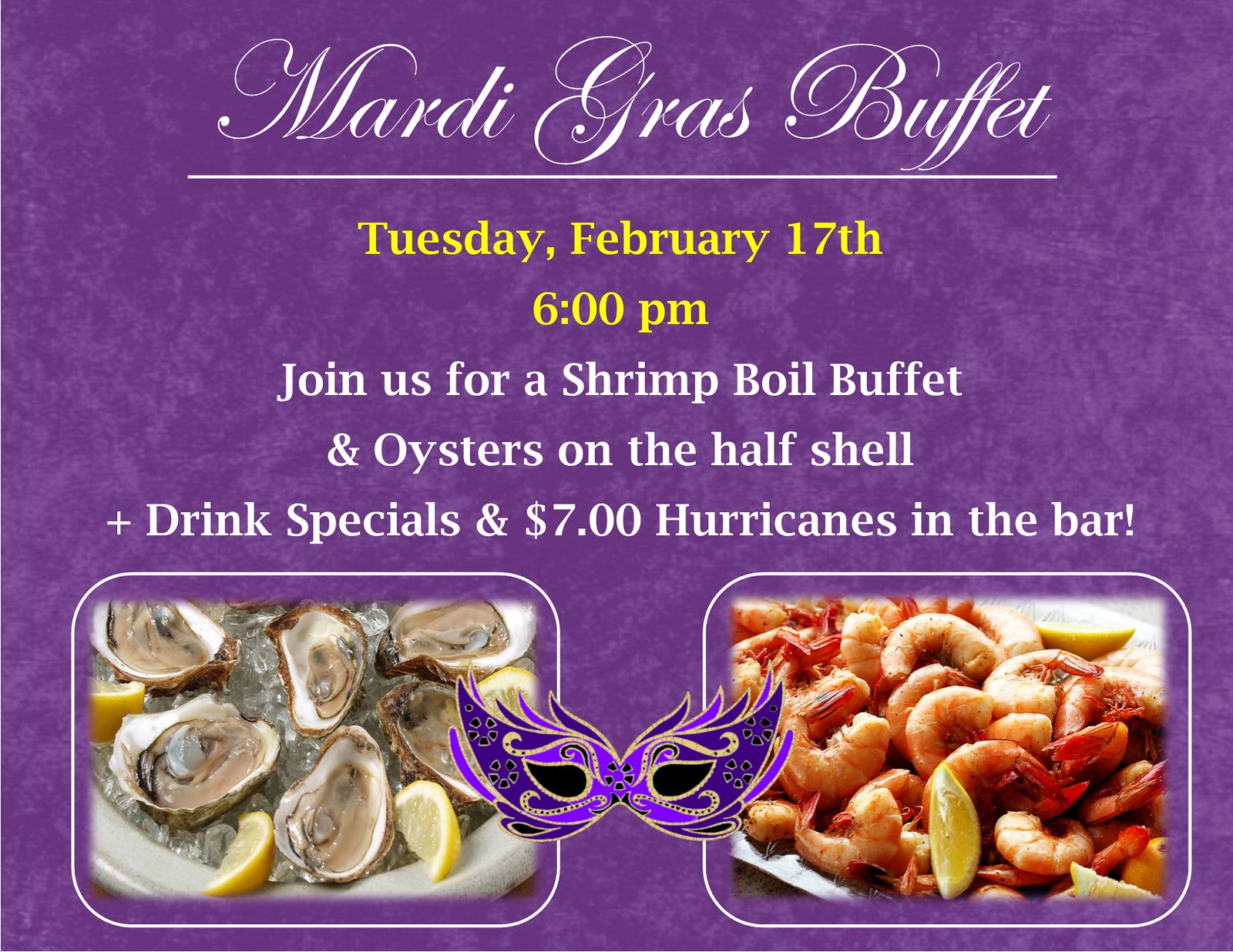This promotional graphic, likely intended for a restaurant's online presence, features a vibrant purple, satin-like background. At the top, elegant white cursive text announces "Mardi Gras Buffet," underlined by a thin white separator. Directly below, bold yellow text details the event date and time: "Tuesday, February 17th at 6 p.m." Continuing in white text, the graphic invites patrons to "join us for a shrimp boil buffet and oysters on the half shell," while also highlighting "drink specials and $7 hurricanes in the bar."

The left side of the graphic showcases a close-up image of oysters on the half shell, neatly arranged on ice within a rounded rectangular border. On the right, another rounded rectangular border frames a generous plate of shrimp, garnished with lemon pieces. Centrally placed between these images is an artistic depiction of a Mardi Gras mask in hues of blue, dark blue, and gold, tying the festive theme together.